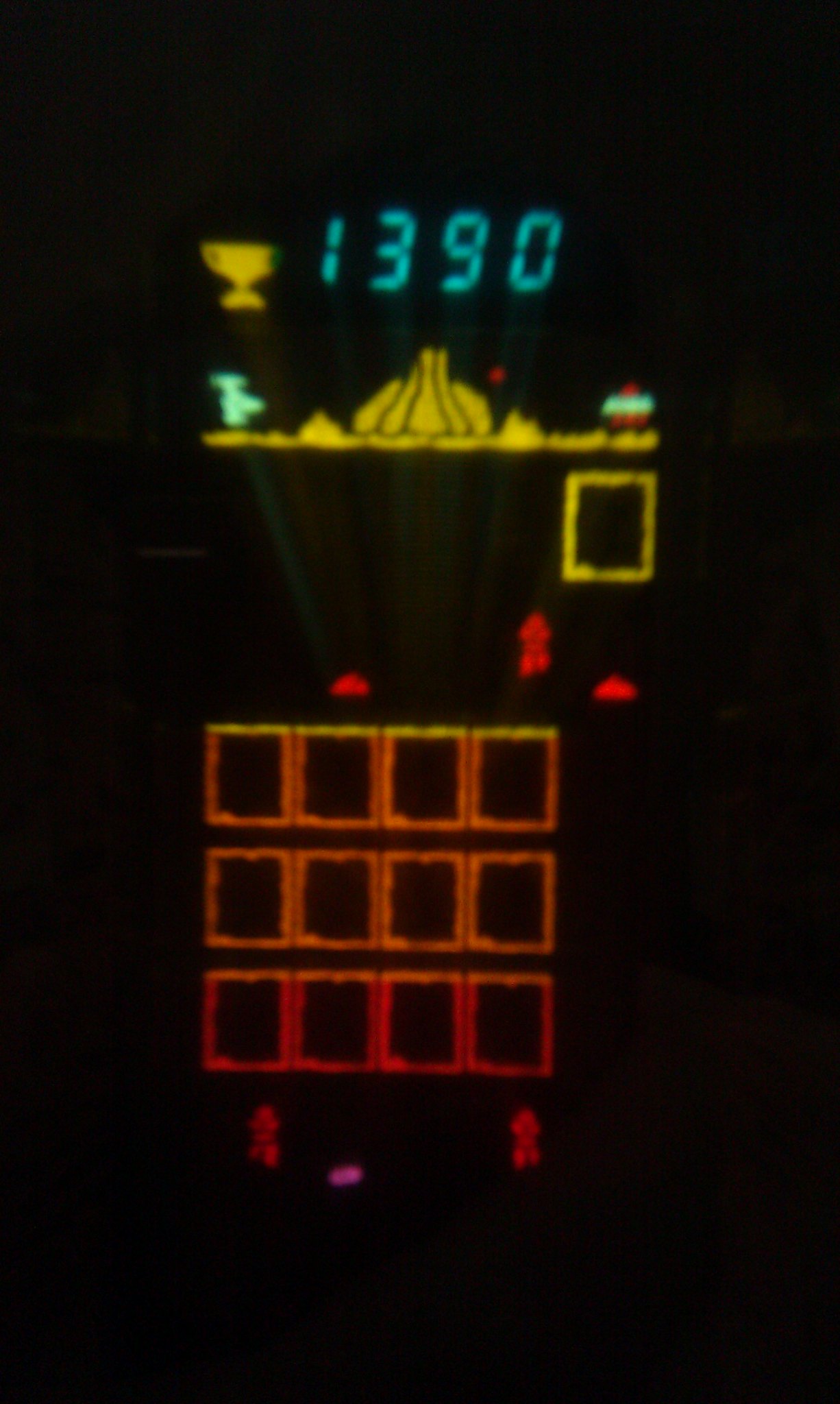This image appears to be a screenshot from a video game. Dominating the scene is a bright yellow trophy, prominently displaying the number "1390." To the trophy's right, there is a green object that is indistinct. Nearby, there is a series of yellow structures that resemble slides. A noticeable red dot aligns with a collection of red and green elements, though their exact nature is unclear.

In the lower section of the image, a yellow square is visible. To its vicinity, there is a vivid red figure resembling a ninja, a red robot, and two additional red entities that appear to be cars. 

There are also eight orange squares, arranged in two rows of four squares each. Below these are four red squares, seemingly organized in a grid pattern. Among these squares, there are two more figures that appear to be red robotic men.